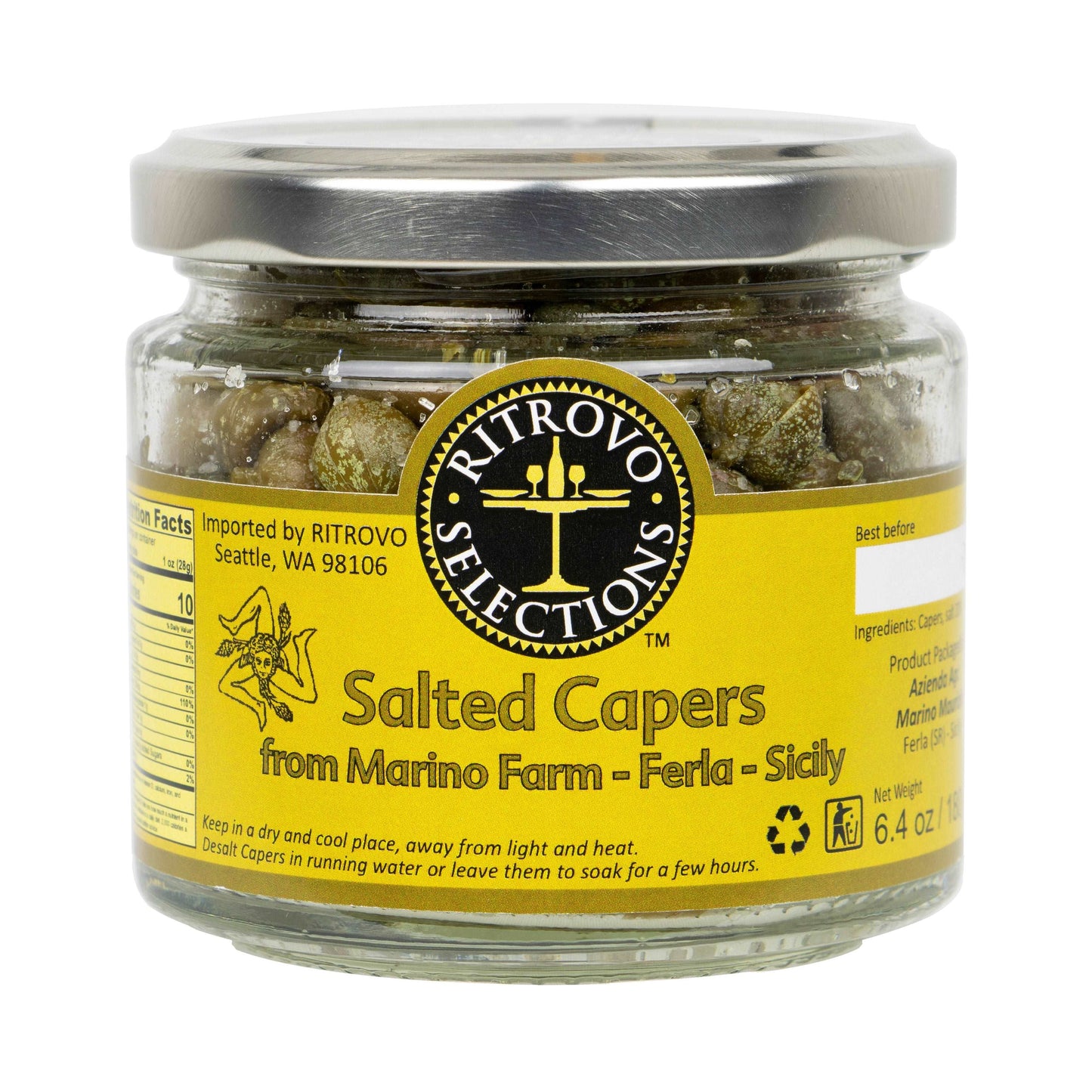The image is a color photograph in square format, showcasing a short, wide glass jar filled with capers. The jar, which has a flat, screw-on silver lid, features a yellow label that wraps around its circumference. Prominently displayed at the top center of the label is a black circle containing white text that reads "Ritrovo Selections." Inside the circle is a line art emblem of a dining table set with a wine bottle and two wine glasses. Directly below the black circle, in gold text, it says "Salted Capers." Beneath this, smaller text reads "from Marino Farm - Ferla - Sicily." The label also includes a recycling emblem with black arrows at the bottom, and advises to "keep in a dry and cool place away from light and heat." The jar's contents, which are small greenish spheres presumed to be capers, are visible through the clear glass. The overall style of the image is photographic representationalism, focusing on realism and product photography against a floating white background.